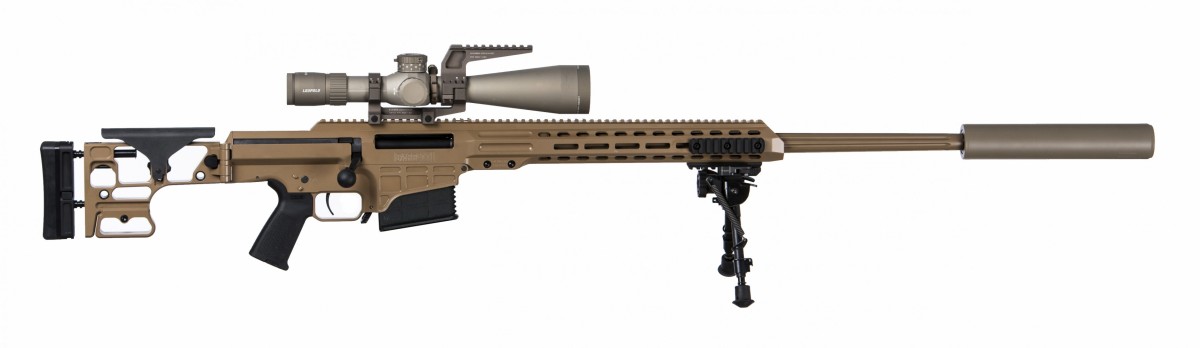This detailed photo showcases a side view of what appears to be an AR-15 rifle. The firearm is secured on a bipod near the midpoint of the barrel for added stability. The gun features a long, brown main body complemented by a gray outer barrel and silencer. It is equipped with a large gray telescopic sight mounted on top, and the trigger handle, bullet cartridge, stock segments, and bipod are all black. Notably, the barrel extends past the bipod and enters a structure that likely protects the user from the barrel's heat before continuing into a suppressor. There are no visible words or logos on the rifle, and it holds a relatively small magazine clip, presumably with a capacity of about eight rounds. The rifle has a sleek combination of brown and gray tones, giving it a sophisticated look.